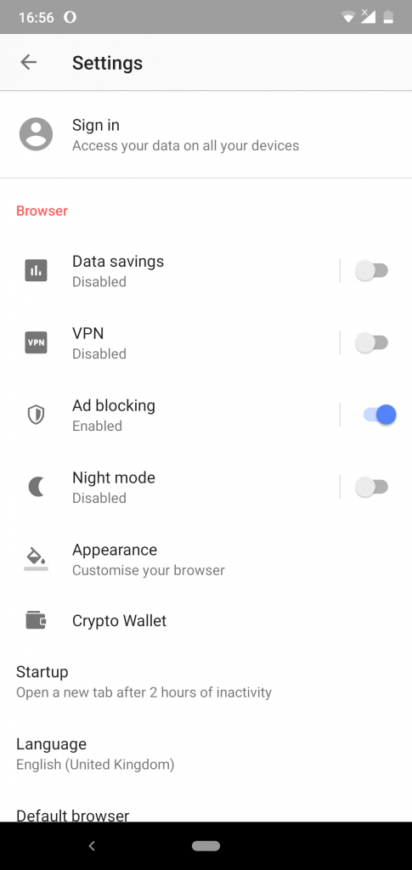This image captures the settings menu of a smartphone's browser application against a light gray background, with details presented in a combination of black and gray text. At the top left, the title "Settings" is prominently displayed in black. Directly below, a user profile section features a gray profile icon on the left and adjacent to it, the text "Sign in" followed by a prompt to "Access your data on all your devices" is written in black.

Further down, the menu displays various settings options starting with "Browser," which is highlighted in red text, while subsequent options are labeled in black. Below "Browser," a "Data Saving" option is shown as disabled, indicated by an off toggle switch in gray. Similarly, "VPN" is also disabled with a gray toggle switch. Contrasting these, the "Ad Blocking" feature is enabled and marked by a blue toggle switch set to on. The "Night Mode" option is disabled, denoted by another gray off toggle switch.

Continuing downward, the "Appearance" section invites the user to "Customize your browser." Further settings include "Crypto Wallet," listed towards the bottom left. Additional details include the "Start up" option set to "Open a new tab after two hours of inactivity," and the "Language" set to "English, United Kingdom." The menu concludes with the "Default Browser" setting, and the bottom of the page is marked by a black bar.